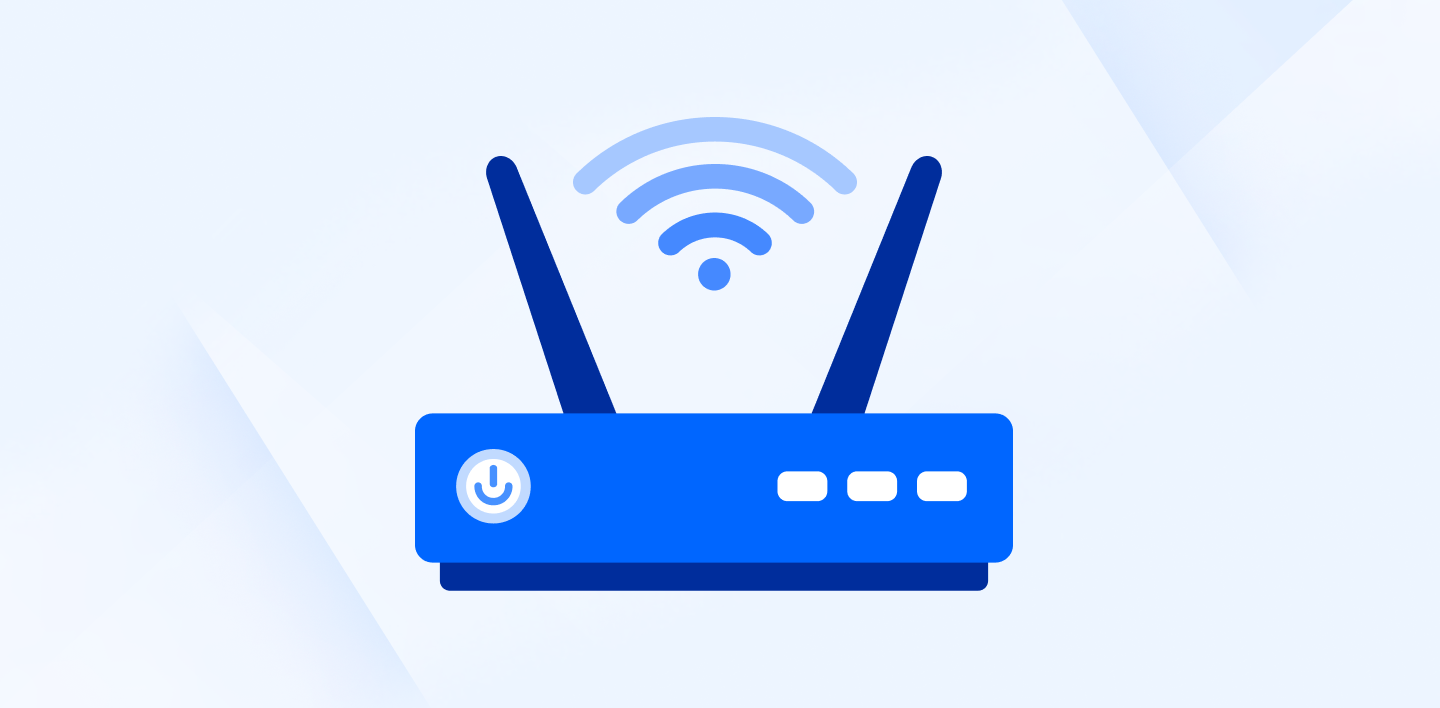This is a simple, stylized drawing of a blue Wi-Fi router. The device features a circular power button with the power symbol on the left side and three white rectangular indicator lights on the right. It has two dark blue antennas emerging from its top, positioned slightly inward from the edges. Between these antennas, the Wi-Fi symbol is prominently displayed, capturing the essence of digital connectivity. The router sits on a dark blue base that is slightly narrower than the main body. The entire image is set against a light blue background, making it predominantly blue except for the white indicators. The overall representation is a clean, iconic portrayal of a Wi-Fi router, symbolizing modern digital communication.